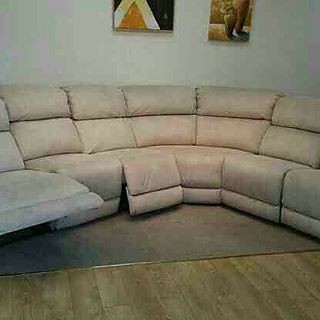This square, slightly overexposed photograph captures an interior home setting, perfect for a shopping site or advertisement. The central focus is a wraparound sectional couch, cropped at both ends, with several seats attached together forming a curve. The couch, which appears to be a light tan or ivory color with a possible grayish tint, is designed with recliners. A section on the far left is fully reclined, while another near the center has its footrest slightly elevated. The couch sits on a dark gray or medium brown thin carpet, placed on a wooden plank floor. The background features a white wall adorned with two artistic, abstract paintings. One image displays yellow and white triangles against a black backdrop, and the other depicts forms resembling vases.